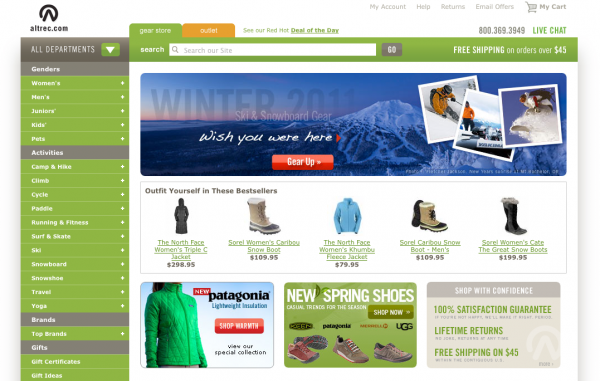The Altrec.com homepage prominently features a vibrant lime green and gray color scheme, reflecting its focus on outdoor wear. The website is meticulously organized into departments categorized by gender, activities, brands, and gift options. Currently highlighted is the "Gear Store" tab, distinctively marked in green, alongside an orange "Outlet" tab. Visitors can easily access the "Deal of the Day," live chat, or contact customer service at 800-369-3949. A notable banner announces free shipping on orders over $45.

Further down, a striking advertisement for the Winter 2011 Ski and Snowboard Gear captures attention, displaying action-packed images of skiers against a majestic mountain backdrop. Various sections feature links to boots and coats priced between $80 and $300. Highlights include an ad for Patagonia's lightweight insulation jackets as well as promotions for spring shoes from renowned brands like Patagonia and Ugg. The bottom right corner reassures customers with a promise of 100% satisfaction guarantee, lifetime returns, and the previously mentioned free shipping offer on orders over $45.